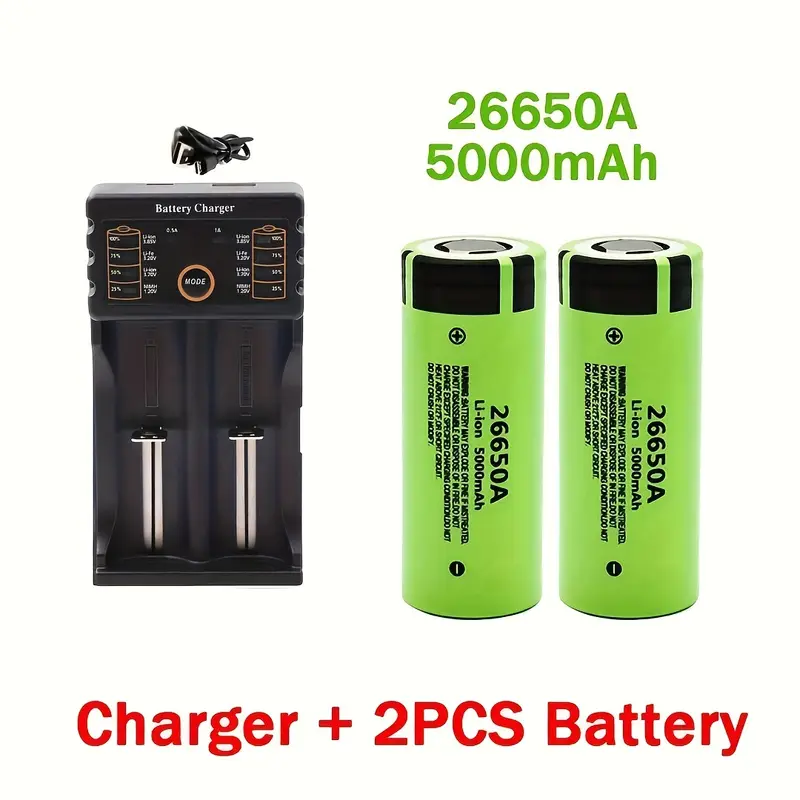This image features a detailed view of a battery charger and two rechargeable lithium-ion batteries. On the left side, a sleek black battery charger, capable of holding up to four batteries, is prominently displayed. The charger includes various settings and modes for optimal charging, with a small cord situated above it for wall connection. To the right, two cylindrical green batteries with black detail and lettering are showcased. These batteries are labeled "ION 26650A, 5000mAh" in black text, with additional model information repeated in green print above. A small black square at the top of each battery includes plus and minus symbols, with a warning label just below. The batteries are arranged on a clean, white background, and at the bottom of the image, bold red text announces "Charger Plus 2 PCS Battery."